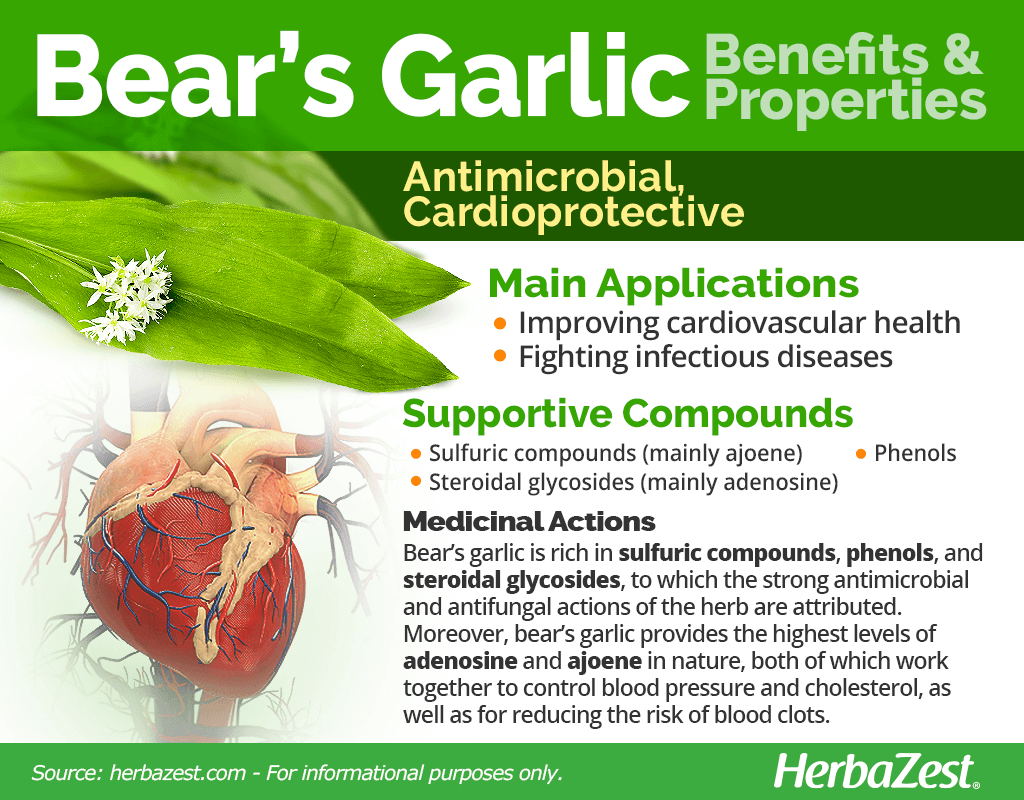This image appears to be an advertisement for Bear's Garlic by Herbazest, likely designed for a magazine. At the top, a green banner with white text prominently displays "Bear's Garlic," and to the right, in lighter green font, it states "Benefits and Properties." Directly beneath this, a black banner with yellow text highlights its "Antimicrobial" and "Cardio Protective" properties.

The upper left of the image showcases leaves with small white flowers. Below the black banner, a white section elaborates on the product with green text stating "Main Applications." It lists bullet points such as "Improving Cardiovascular Health" and "Fighting Infectious Diseases." This section is followed by the phrase "Supportive Compounds," detailing constituents like sulfuric compounds, phenols, and steroidal glycosides, which are identified for their health benefits.

To the left in this section, an image of a heart symbolizes cardiovascular health benefits. Continuing below, black text outlines "Medicinal Actions," explaining that Bear's Garlic is rich in sulfuric compounds, phenols, and steroidal glycosides, which contribute to its antimicrobial and antifungal properties. It also mentions that Bear's Garlic provides high levels of adenosine and ajoene, compounds that help regulate blood pressure, cholesterol, and reduce blood clot risks.

At the bottom, a smaller green banner with white text notes "Source: herbizest.com for informational purposes only." Adjacent to this on the right, "Herbazest" is prominently displayed in larger text, reiterating the brand name.